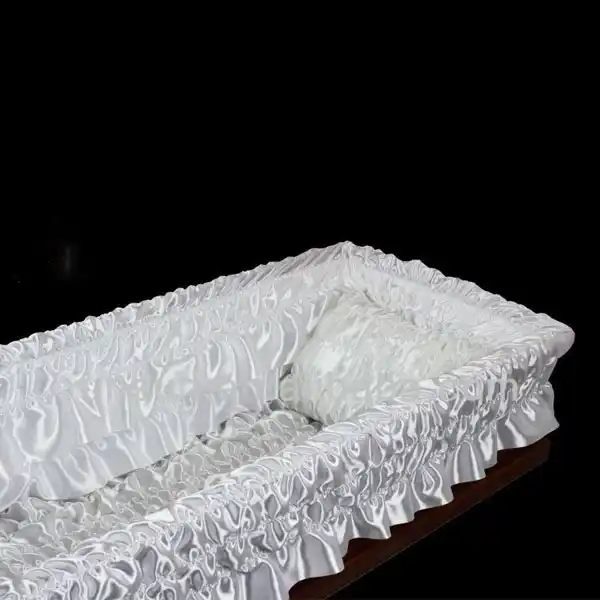In the image, a casket is prominently displayed at a diagonal angle. The top of the casket is opened, revealing a luxurious white sheet draped inside. The sheet has a silky texture, exuding a shiny and pristine appearance. Atop the sheet rests a pillow made from the same silky material, equally soft and shiny. This scene suggests the setting of a funeral service. The base of the casket, visible at the bottom right corner, is crafted from dark brown wood, adding a somber touch. The background is predominantly dark, with a small, reflective glass object visible on the left side above the casket.